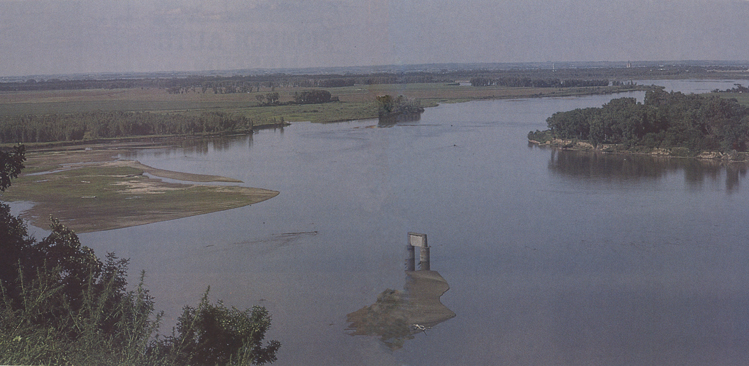The image depicts a gray and grainy scene of a broad, murky river stretching across its entire width, likely scanned from an old newspaper, suggested by the faint text visible in the background. The setting is gloomy and hazy, enhancing a sense of bleakness which might be due to either the weather or the poor quality of the photo. The river is full, with its expanse giving way to a mix of overgrown green patches and patches of mud. 

In the foreground, to the bottom left, some trees are visible, providing a touch of greenery against the overall desaturated tone. A small, verdant island is situated towards the middle or top right, densely covered with foliage and adding a hint of mystery to the scene. The middle of the river features what appears to be a sign or possibly some debris, partly submerged and indistinct. In the distance, a faint, ambiguous outline could be mountains but remains indistinct due to the image's graininess. The mixture of browns and murky water creates a somber yet intriguing landscape.